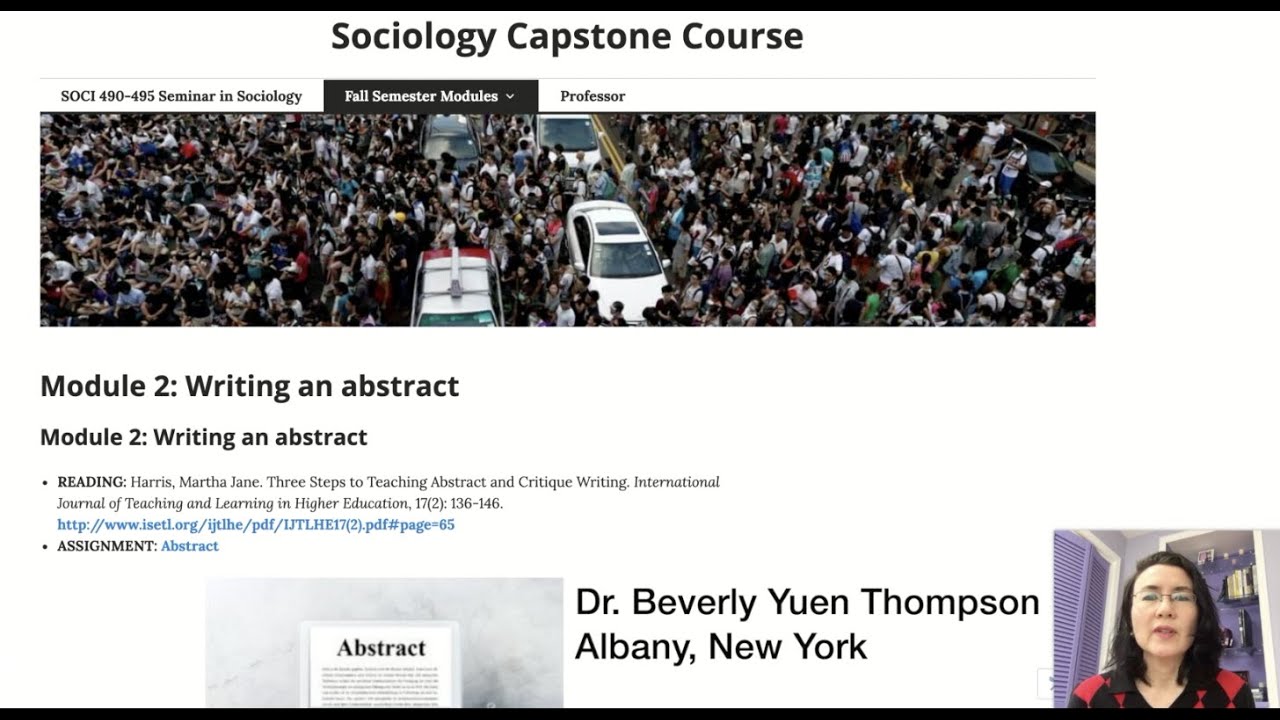A screen capture from a web page titled "Sociology Capstone Course" displays a navigation ribbon at the top with three selectable items. The first, on the left, is labeled "SOCI 490-495 Semester in Sociology." The middle tab, "Fall Semester Modules," is highlighted in black. The rightmost tab is labeled "Professor."

Below the navigation ribbon, there's an aerial photograph of a bustling street crowded with people and some vehicles. Beneath the image, on the left side, the text reads, "Module 2: Writing an Abstract." It continues with a reading assignment: "Harris, Martha Jan. ‘Three Steps to Teaching Abstract and Critique Writing.’ International Journal of Teaching and Learning in Higher Education, 17(2), 136-146," along with a web page link. There is also an "Assignment: Abstract" section.

On the right side at the bottom, it mentions "Dr. Beverly Wood Thompson, Albany, New York," accompanied by a portrait of her. She appears to be an Asian woman in her early 40s, wearing glasses.

This screen capture detailedly showcases the information for the "Writing an Abstract" module in the fall semester of the Sociology Capstone Course, along with a visual reference of Dr. Beverly Wood Thompson.